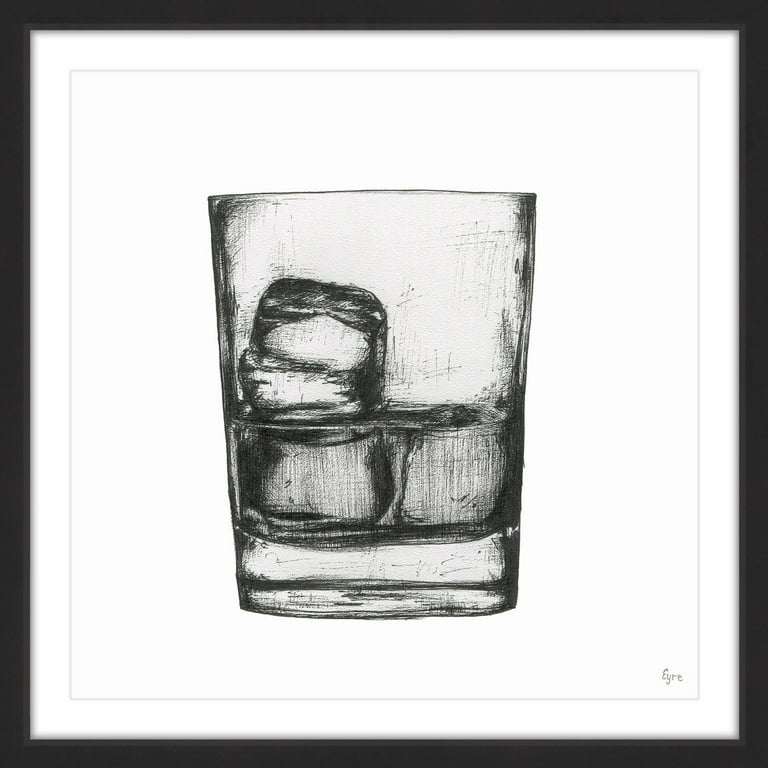The piece is a black, white, and gray pencil drawing of a glass tumbler, about one-third filled with water. The liquid fills the glass just above two ice cubes submerged at the bottom, with another ice cube protruding above the water’s surface on the left. The sketch effectively employs shading to depict the varying textures and to convey the three-dimensional form of the glass and ice. The drawing is encased in a sophisticated multi-layered frame: starting from a white background, a gray square surrounds the image, followed by a white border, and finally encased by a thick black frame. The simplicity of the scene stands out against the plain white background with no additional objects to distract from the central subject. It features the artist's signature, "EYRE," in the bottom right-hand corner. The artwork aligns with a modern minimalist style, capturing stark details through precise pencil strokes and shading.